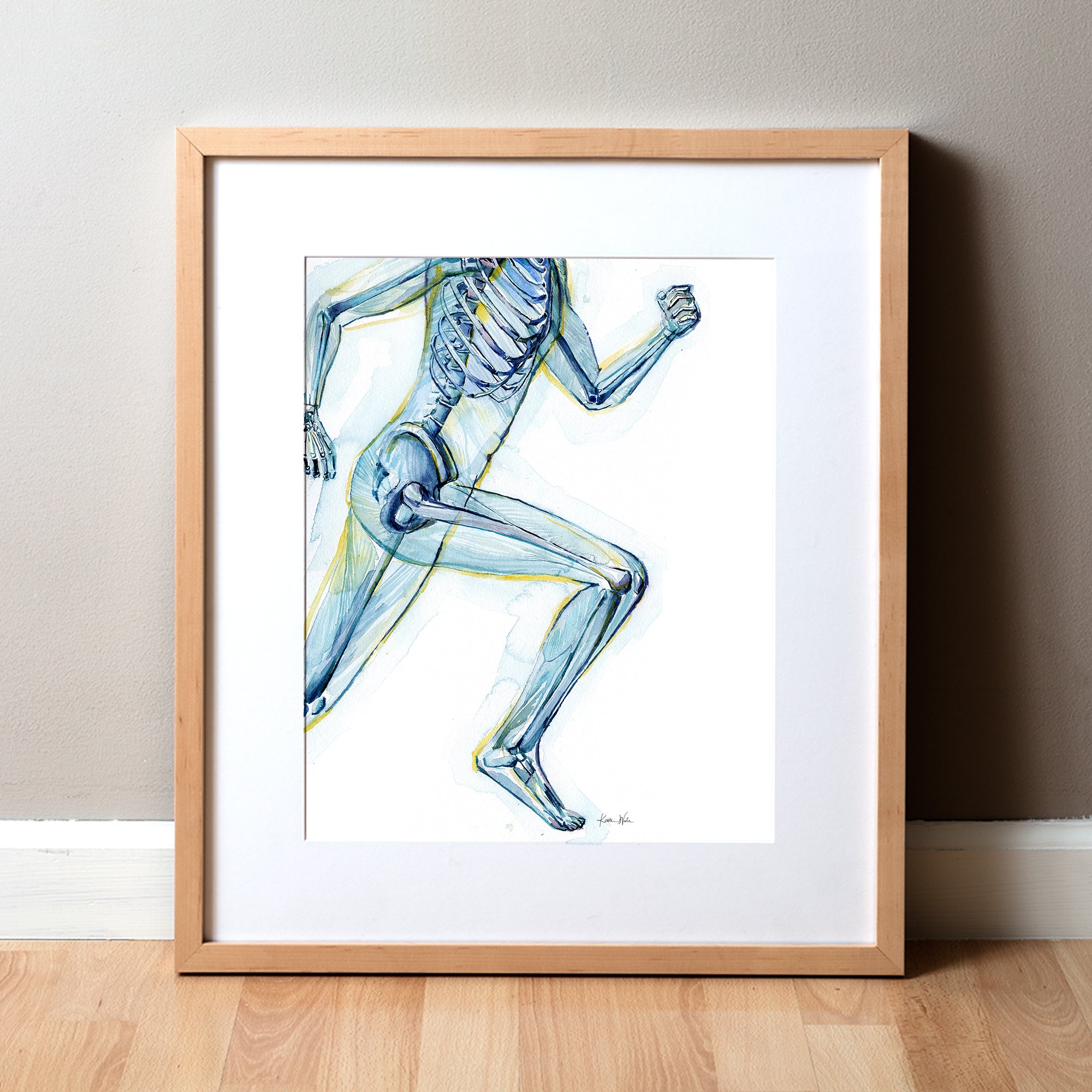This photograph showcases a detailed x-ray-style drawing of a human figure mid-stride, encased in a basic light brown wooden frame with a white mat border. Resting on a pale hardwood floor next to a white baseboard and a grayish wall, the artwork predominantly features hues of blue, yellow, and green, with hints of black. The side profile captures the dynamic motion of running, where the right leg and left arm push forward and the left leg and right arm trail behind, some parts extending slightly out of frame. Visible are the person's skeleton and the faint outline of their translucent skin. Positioned by the front foot's base is an artist's signature, though it's unreadable. The drawing occupies approximately the first third of the canvas against a stark white background, emphasizing the centrality and motion of the skeleton runner.